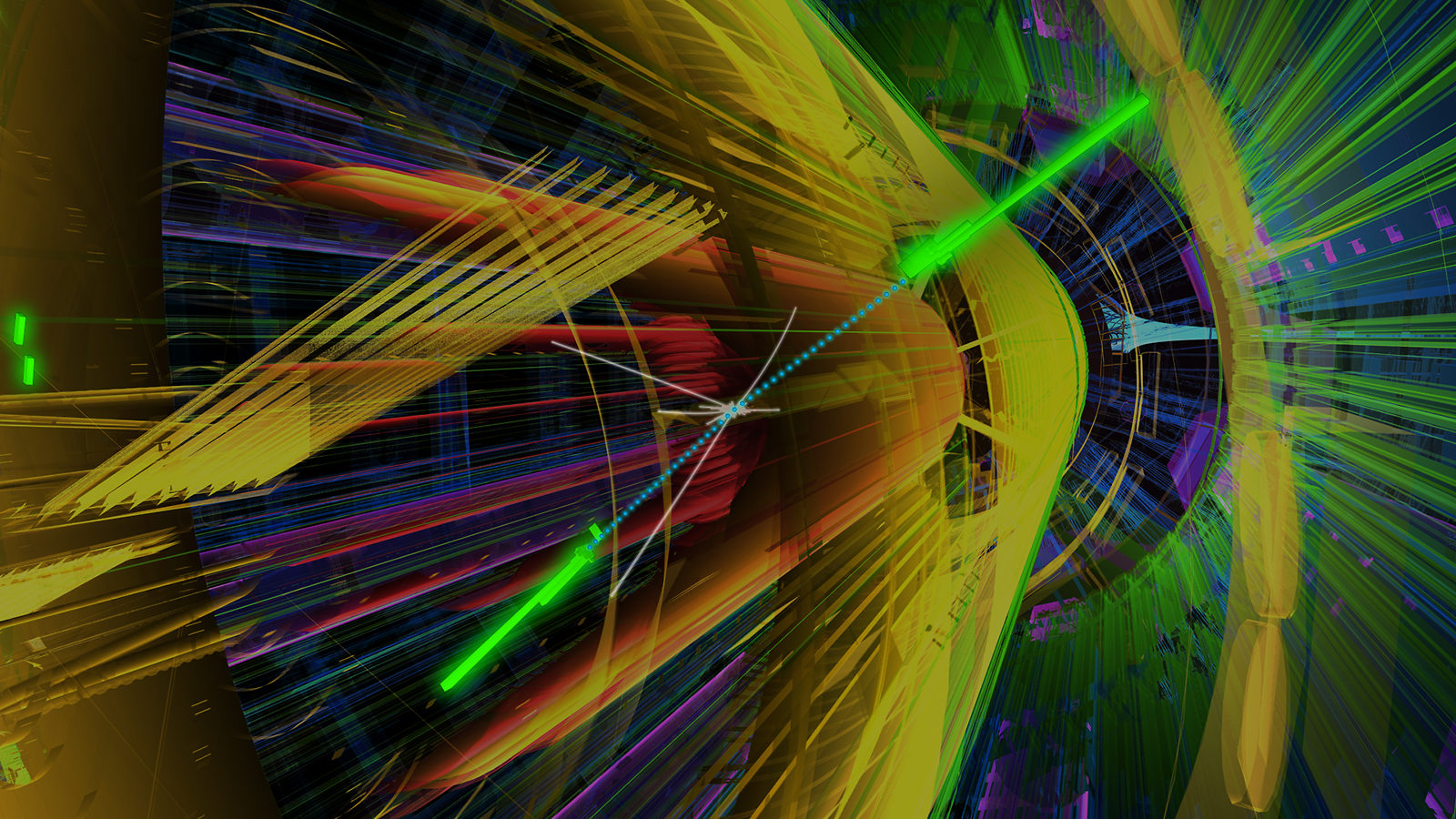This image features a vibrant, abstract scene composed of countless laser-like streaks of light, converging towards the center in a rectilinear landscape format. The image, which appears man-made and possibly digitally crafted, bursts with dynamic neon colors including yellow, red, blue, purple, pink, green, orange, black, and gold. These straight lines create a sense of motion and energy, similar to the dispersal pattern of flames from a rocket's launch. Prominent among the streaks are two luminescent green lines connected by a blue, chain-like light. The overall aesthetic conveys an impersonal, futuristic technology, with a visual impression of colored lights traveling or dispersing away from the viewer's perspective. The scene evokes an impression of a light show or a complex graph, characterized by its vivid hues and abstract geometric precision.